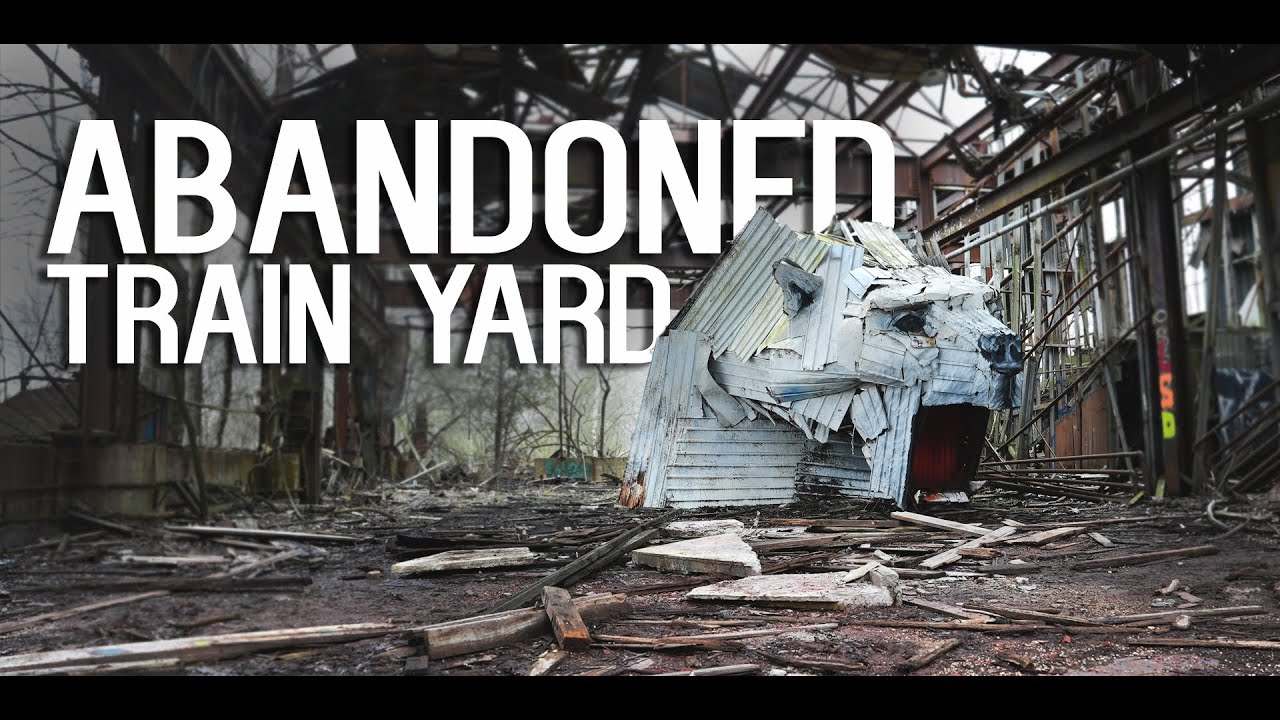The image depicts a desolate and dilapidated outdoor area, identified by bold, white block letters at the top left as an "abandoned train yard." Dominating the center of the scene is a tattered white structure that appears on the verge of collapse, surrounded by scattered debris. The floor is strewn with broken and soiled wooden pieces, intermingled with rusted, brown metallic beams and wire framing. The ground itself is a brownish-gray shade, contributing to the overall sense of decay. Notably, on the right side of the image, the letters "LSD" are spray-painted in vibrant colors, with the 'L' in red, 'S' in orange, and 'D' in green, adding a stark contrast to the bleak setting. The area exudes the atmosphere of a ruined, abandoned yard.